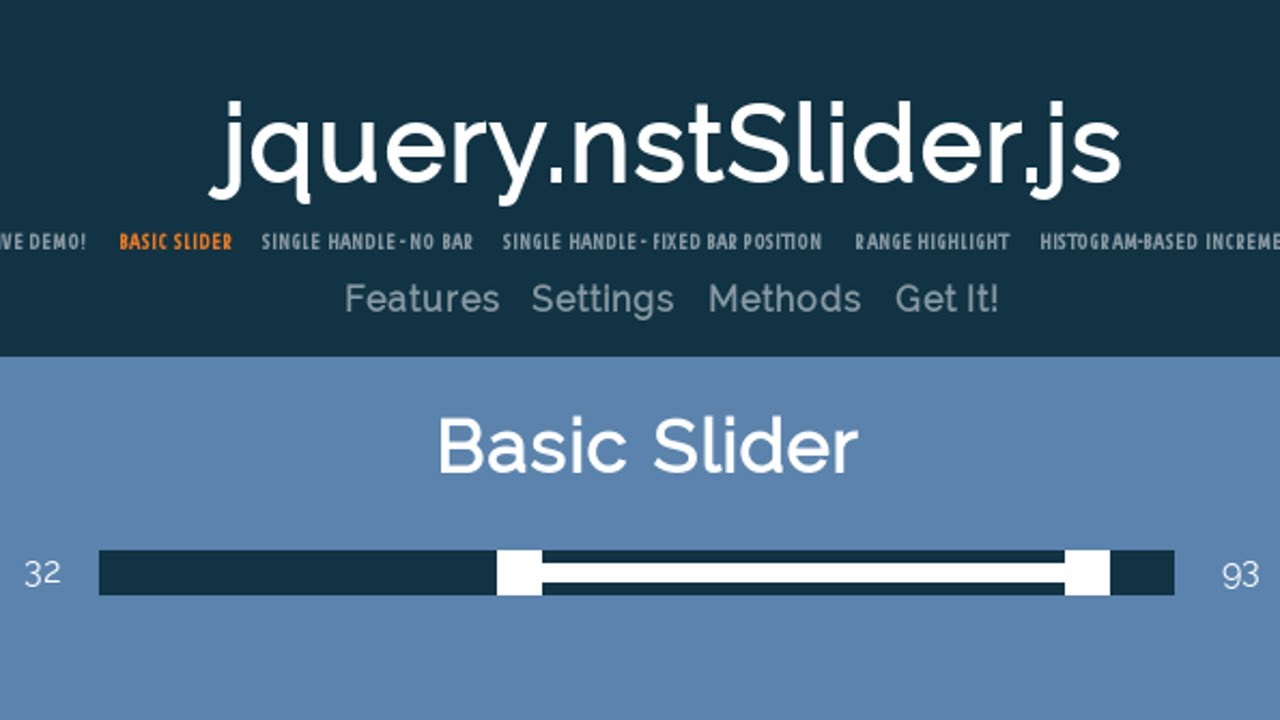The image features a background gradient that transitions from dark blue at the top to light blue at the bottom. At the upper portion of the image, the text "jquery.nstslider.js" is prominently displayed, followed by the word "Demo" beneath it. A section titled "Your Basic Slider" is highlighted in orange and lists several slider features: "Single Handle," "No Bars," "Single Handle with Fixed Bar Position," "Range Highlight," and "Histogram Based Increments."

Further down, the categories "Features," "Settings," "Methods," and "Get It" indicate additional functionalities or navigation options.

In the lighter blue bottom section, the text "Basic Slider" is presented in white print. On the left side, the number "32" is shown. Adjacent to it, a black rectangular box frames a white slider that moves horizontally between the black edges. At the end of the slider, a square marker is displayed with the number "93" to its right, also in white. This entire component rests against the light blue background, illustrating a basic slider mechanism where a black line is overlaid with a white slider part.